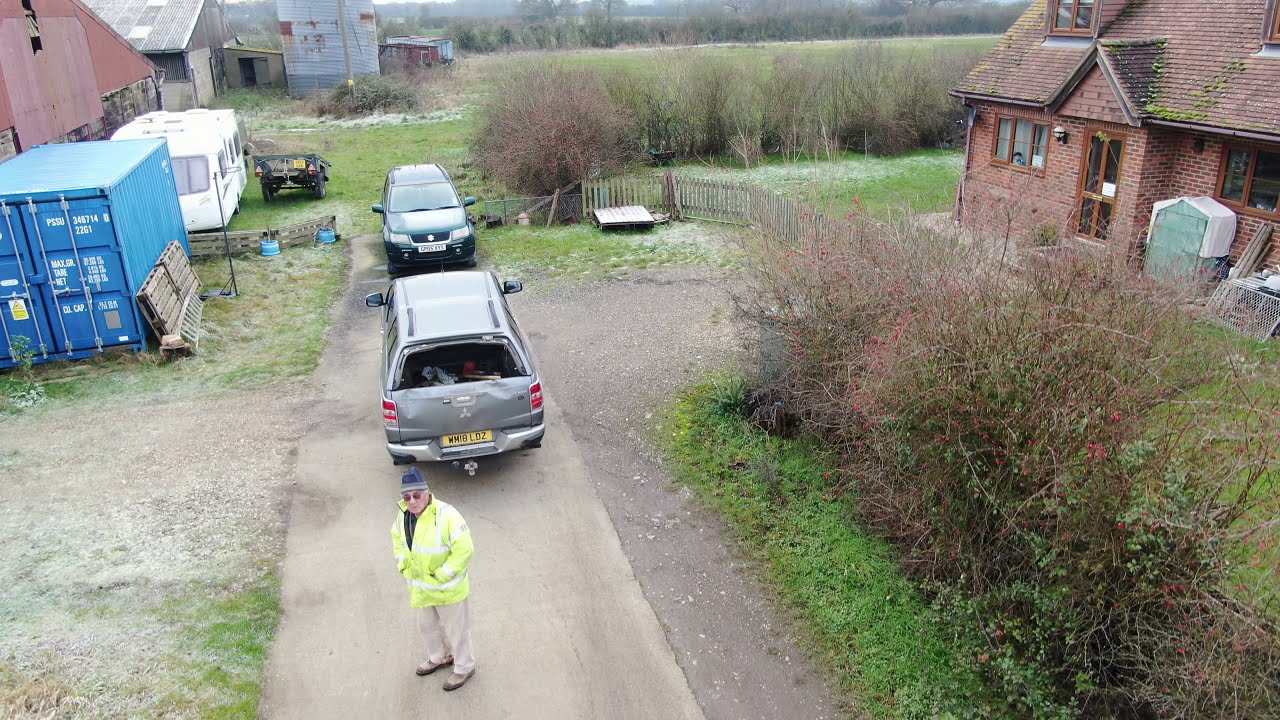This landscape-oriented, color photograph captures an aerial view, possibly taken by a drone, of a rural front yard and driveway of a two-story red brick house with a brown shingle roof. The house is surrounded by a large grassy area with trees and various hedges. In the front yard, distinct details are visible, including a tall, wooden picket fence and a pebbled pathway composed of stones and rocks.

Central to the image is a man, positioned near the bottom left corner, standing on a concrete driveway. He is dressed in a blue hat, sunglasses, a bright yellow jacket typical of a city worker, a black shirt underneath, beige trousers, and khaki shoes. Behind the man is a silver truck with several dings on the back and a European tag, while in front of the truck, facing towards the viewer, is a bluish-green, turquoise Honda CRV.

Across the street from the driveway, there is a large blue shipping container and a white RV parked alongside a shed with a striking red roof. Additional sheds and outbuildings are visible nearby, enhancing the rural ambiance of the scene. The landscape includes more grass, trees, hedges, and bushes that envelop the setting, suggesting a serene countryside atmosphere.